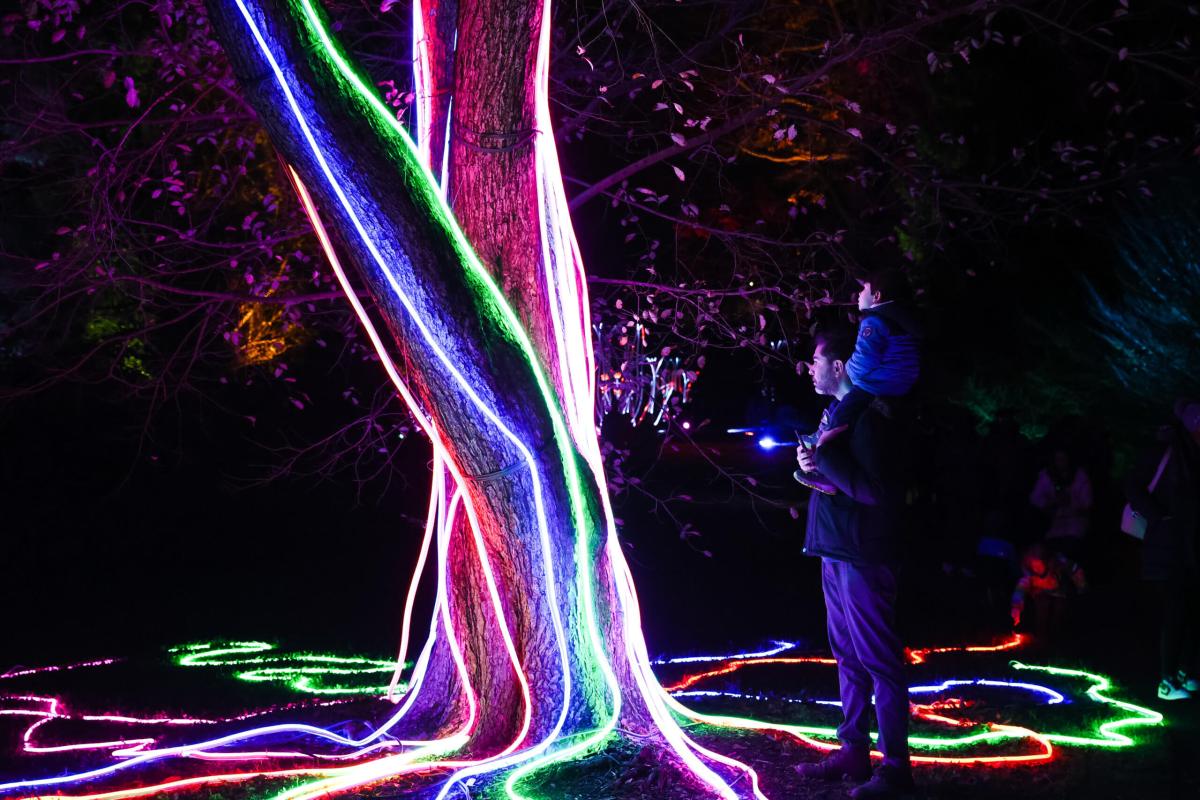In this captivating night-time photograph, a father stands with his child perched on his shoulders, the little one bundled in a blue coat and possibly donning a black hat. They are positioned to the right, gazing at an enchanting scene before them—a tree adorned with an array of vibrant neon lights. The luminous display includes striking blue, green, red, pink, and purple colors that cascade down the trunk and artistically swirl around the ground, creating a mesmerizing spectacle. The background reveals dark silhouettes of branches and leaves, adding depth to the scene. This enchanting setting, with its electrifying ambiance, hints at an outdoor light show, perhaps in a forest, a museum, or a theme park-like environment, evoking a sense of wonder and shared discovery.